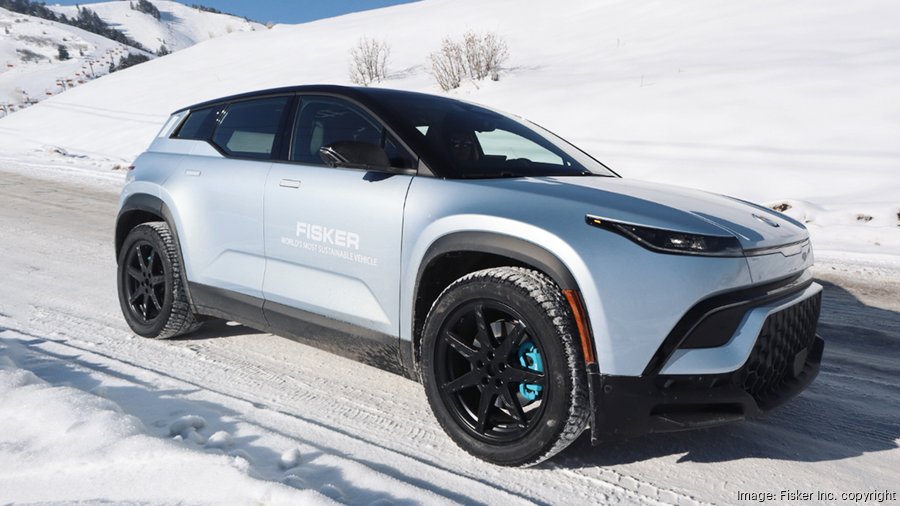This landscape-oriented photograph captures a compact pale blue car with large snow tires, driving on a snow-covered roadway in the mountains. The car, a four-door with a black top and thin headlights, features white text on the door reading "Fisker" along with the phrase "the world's most sustainable vehicle" in smaller letters. In the foreground and background, substantial snowfall is evident, with a couple of brown bushes peeking through the snow. The mountainous backdrop, also blanketed in snow, adds depth to the scene. The car is traveling toward the right side of the image, and though difficult to discern, the driver wearing sunglasses appears to be a woman. In the bottom corner, the text "image Fisker Inc copyright" is faintly visible. The emphasis of the photo remains on the car navigating through the pristine, snowy surroundings.